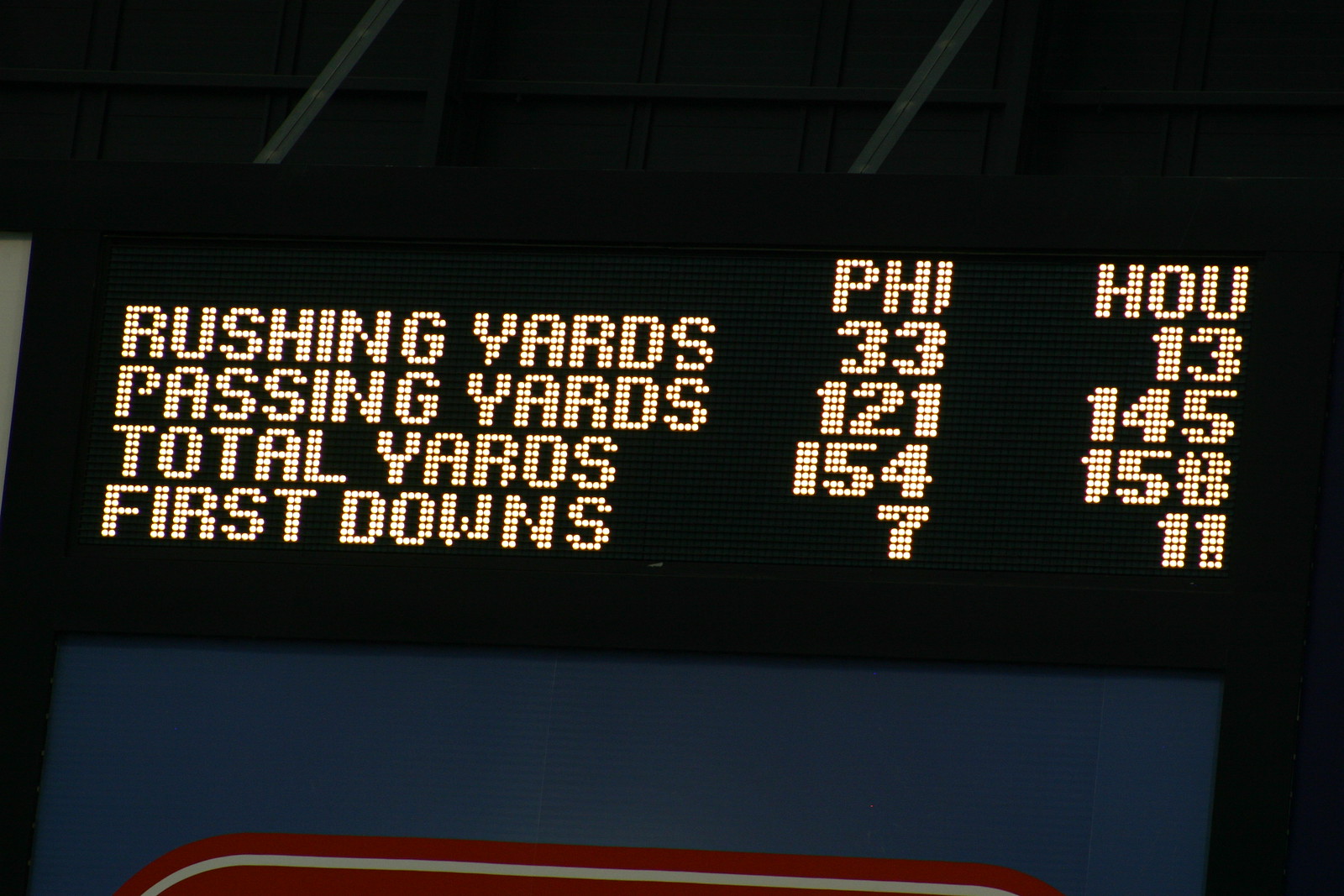The image presents a close-up view of a digital football scoreboard, displaying comparative statistics between two teams: the Philadelphia Eagles (PHI) and the Houston Texans (HOU). The scoreboard features a black, digital display with yellowish dotted text. The left side of the board lists statistical categories: rushing yards, passing yards, total yards, and first downs. The corresponding statistics for each team are shown in two adjacent columns labeled PHI and HOU.

For rushing yards, Philadelphia has 33, while Houston has 13. In passing yards, Philadelphia records 121 compared to Houston's 145. The total yards amount to 154 for Philadelphia and 158 for Houston. Lastly, the first downs are noted as 7 for Philadelphia and 11 for Houston, though one light is missing in the digit for Houston's first downs.

Below the statistical display, partially visible, there is a blue square with a red bar above it, accompanied by two gray lines extending upwards, though this section is cut off. The overall display is set against a dark, solid-colored background that appears dark gray to brownish.